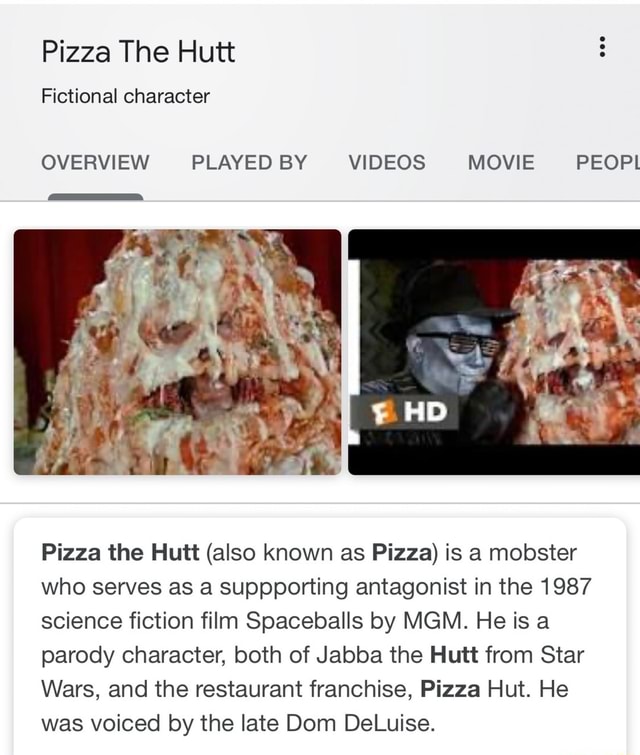Pizza the Hut, also known simply as Pizza, is a fictional character and mobster who appears as a supporting antagonist in the 1987 science fiction comedy film "Spaceballs," produced by MGM. Parodying both Jabba the Hutt from Star Wars and the Pizza Hut restaurant franchise, Pizza the Hut is portrayed as a grotesque, anthropomorphic pizza with gooey, dripping cheese and a menacing demeanor. Voiced by the late Dom DeLuise, this character adds a comedic yet villainous element to the film's plot.